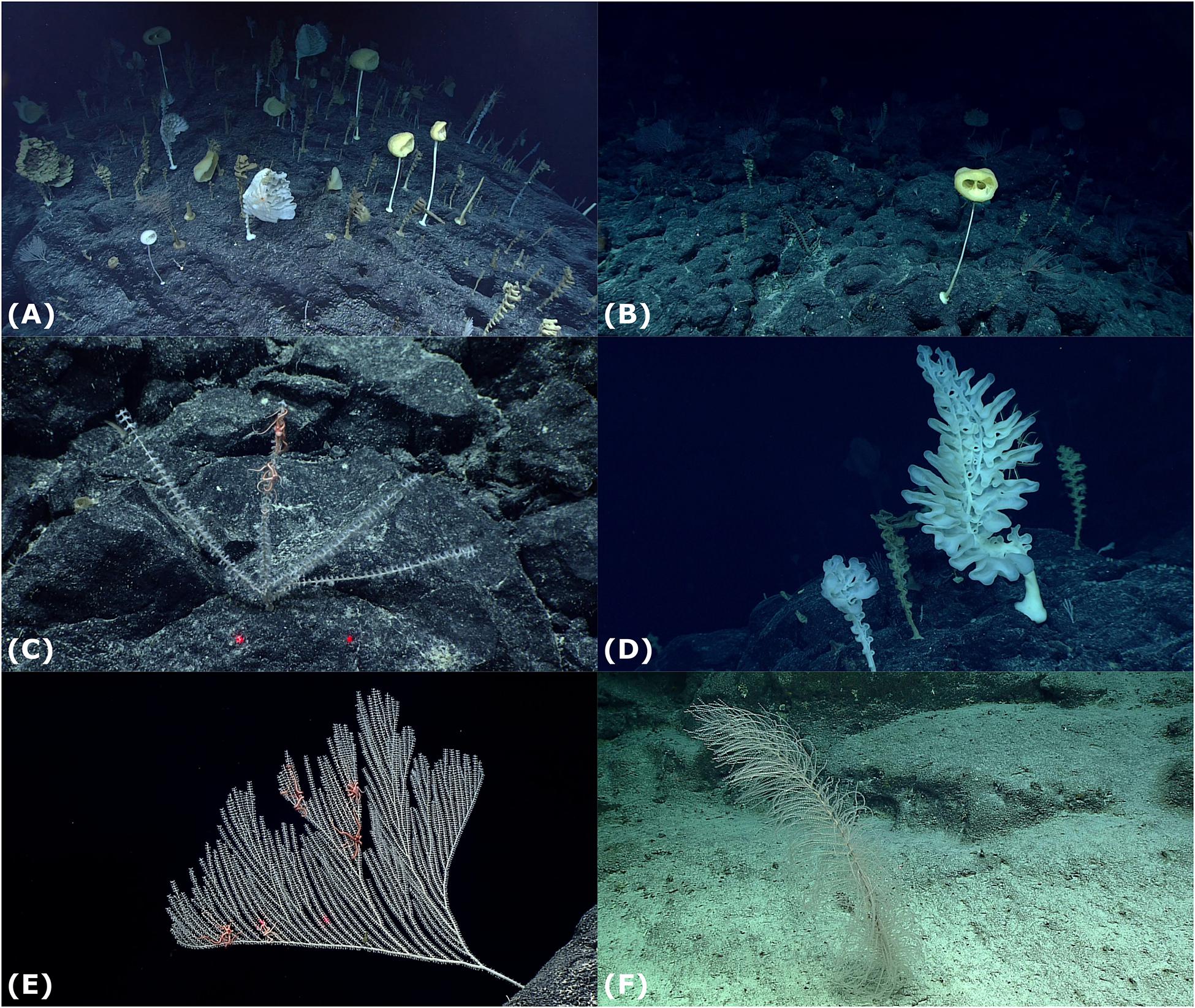The image consists of six distinct underwater photographs arranged in a grid, labeled A through F. Each quadrant reveals unique aspects of marine life, showcasing the diversity of underwater ecosystems. In quadrant A, there's a subdued scene of a coral reef featuring a yellow-green-blue sea anemone. Quadrant B presents a darker and sparser coral reef environment similar to A, but with fewer sea anemones. Quadrant C displays a black rock adorned with moss and a striking blue, thread-like plant. In contrast, quadrant D captures a deep water setting with translucent, ghostly blue organisms resembling floating organs. Quadrant E is predominantly pitch black, showcasing a beige, woven tree branch-like structure, evocative of underwater foliage. Finally, quadrant F illuminates a sandy ocean floor bathed in more light than the other quadrants, highlighting a beige, stringy plant. Together, these images portray a fascinating progression of underwater plant and plankton life, each quadrant offering a glimpse into different marine habitats and their intricate details.